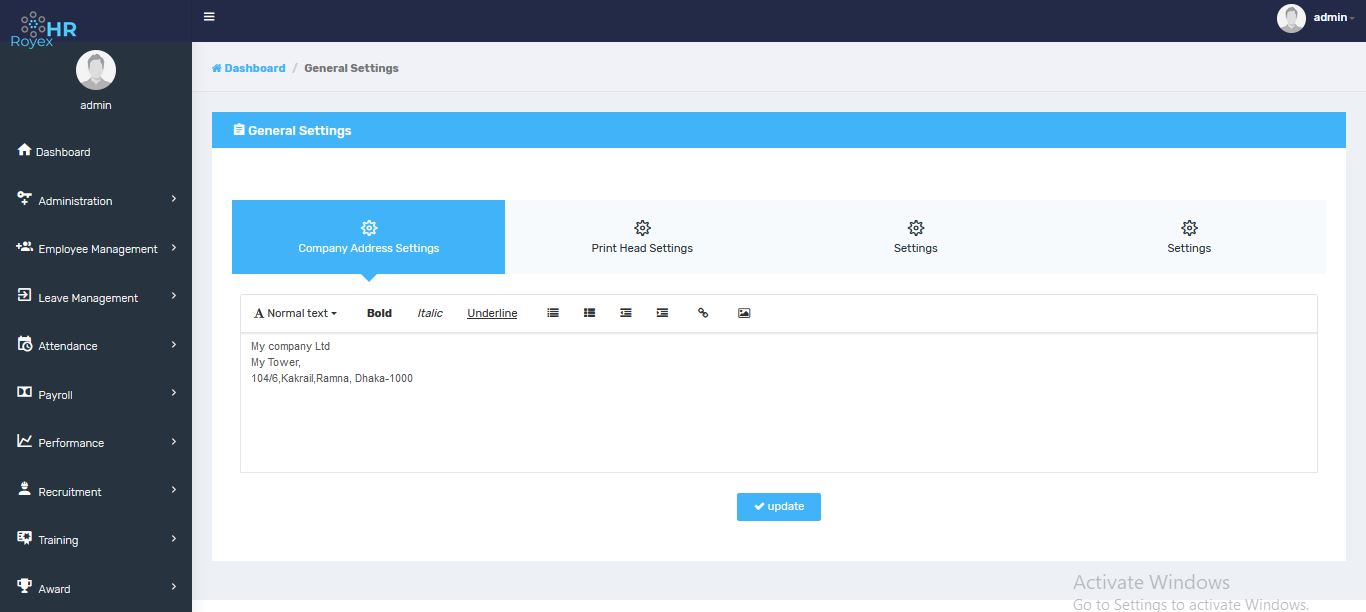**Detailed Caption:**

This image is a screenshot of a website interface displaying an HR management portal. The top of the interface features a light blue snowflake-like symbol beside the letters "HR," indicating the theme of the platform. Running down the left sidebar, which is highlighted in black, are navigation options including: Dashboard, Administration, Employee Management, (unreadable) Management, Attendance, Payroll, Performance, Recruitment, Training, and another option starting with 'A'. 

Within the sidebar's 'Administration' section, users can see a circular icon with the label "Admin" and another identifier that seems to be "RoyX" or "RoyFx." The main content area of the webpage is currently showcasing 'General Settings' with a light blue header bar that reads "Dashboard" and a gray bar that says "General Settings." 

Beneath this header, a box with a blue banner titled "General Settings" offers four options: Company Address Settings, Printhead Settings, and two instances simply labeled "Settings." These options likely allow users to configure various aspects of the platform. At the bottom of this settings box, there's a prominent blue button labeled "Update," allowing users to save their changes.

This detailed view helps in managing and navigating the different functionalities of the HR system effectively.